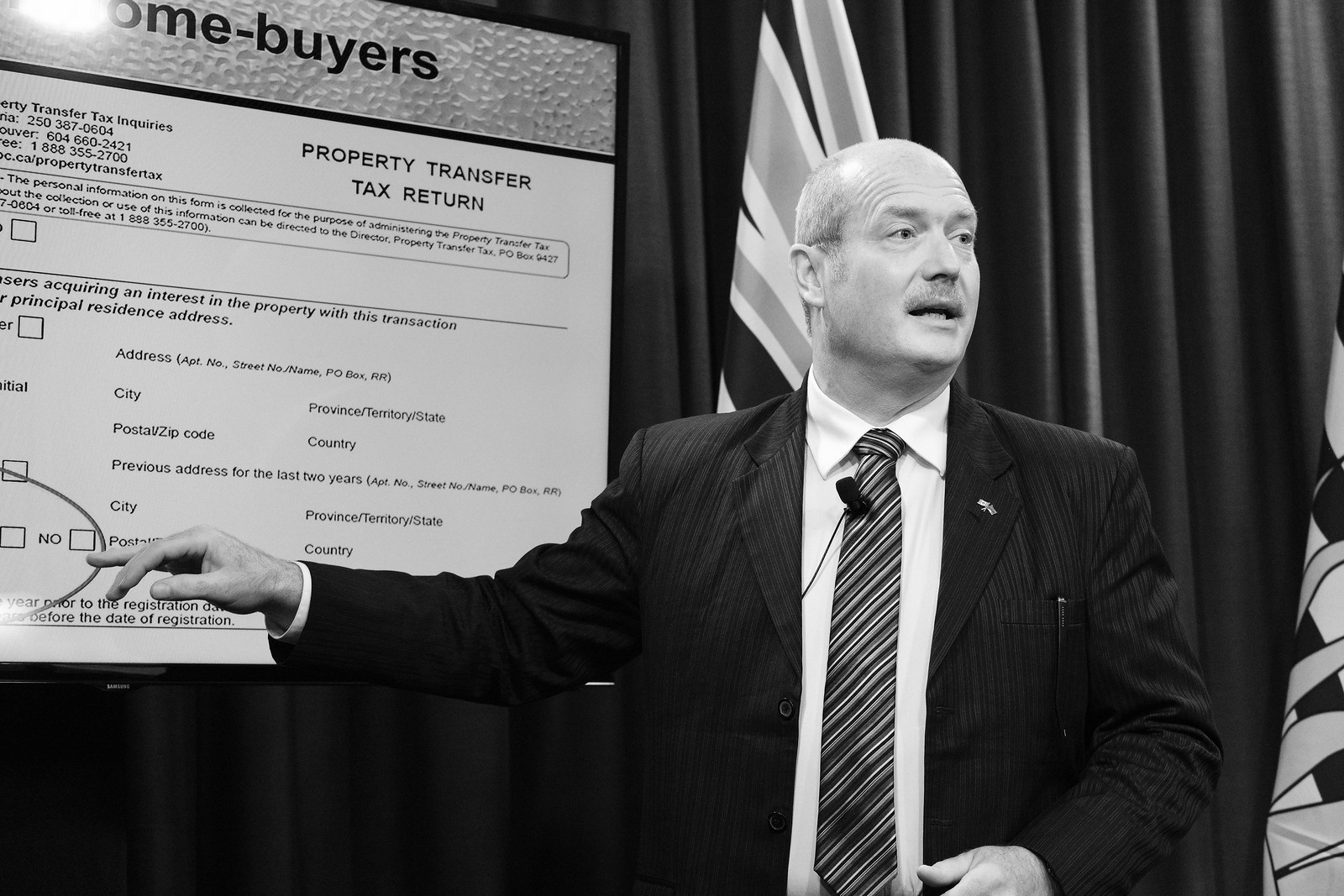In this black, white, and gray photograph, a serious, bald man is giving a speech or presentation, presumably about home buying and property taxes. Standing on a stage set against a backdrop of draped curtains and two flags, he is dressed in a dark, pinstripe suit with a complementary striped tie, and a white button-down shirt. He has a mustache and is equipped with a microphone. With his right hand, he points toward a screen displaying text that includes phrases like "homebuyers," "property transfer tax return," "address," "city," "postal/zip code," and "country." The displayed information is likely related to the procedural details of buying a home. The rest of the screen's small text is illegible due to its tiny size and the distance from the viewer. The monochromatic palette emphasizes the official and focused atmosphere of the event, though the presence of "red" curtains, inferred from the black and white image, adds a visual anchor to the setting. The audience is not visible in the photograph, keeping the emphasis entirely on the speaker and the content of his presentation.